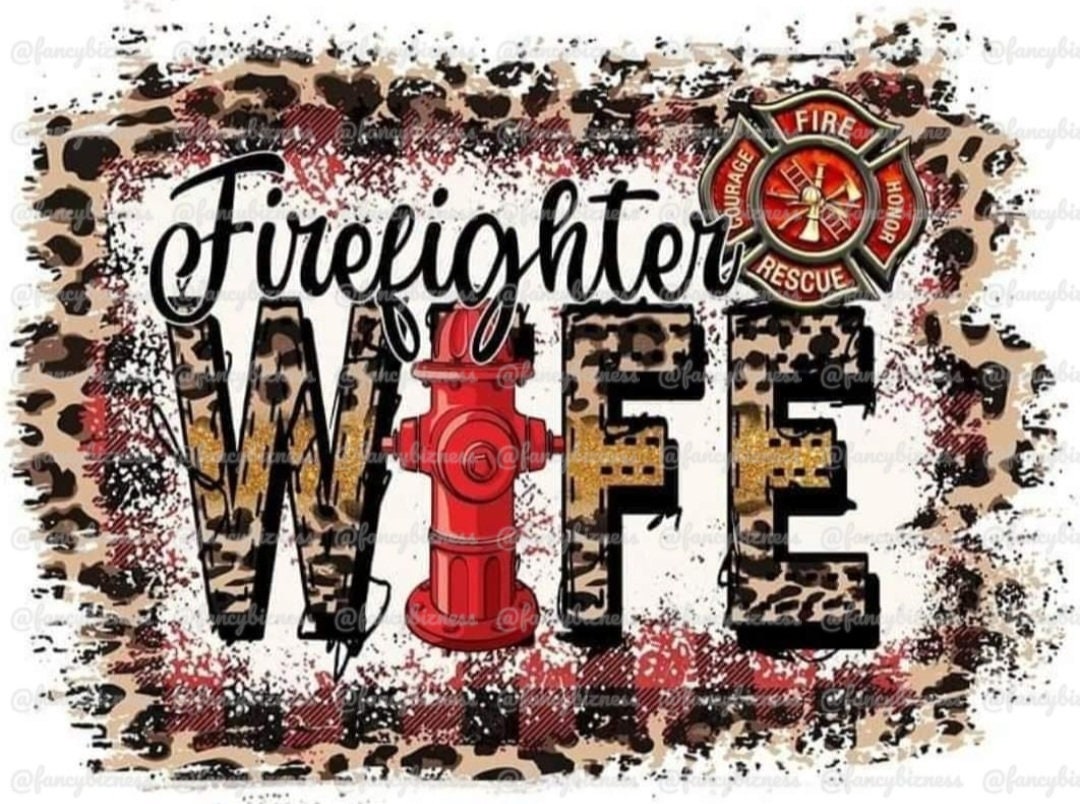The image features a white background with the phrase "Firefighter Wife" prominently displayed. "Firefighter" is written in elegant black cursive letters at the top, while "Wife" is emphasized below with the letters W, F, and E in a large, eye-catching leopard print font. The I in "Wife" is creatively replaced by a red fire hydrant. The piece is framed by a border featuring red and black splotches and paint splatters, surrounded by a speckled leopard print design. In the upper right corner, there is a detailed fire department emblem. The emblem, resembling a red seal, includes the words "Fire Rescue" and features various firefighting equipment within its central circle, flanked by the words "Courage" and "Honor" on either side. This visually striking artwork is likely to be seen on a social media post, celebrating the pride and bravery associated with being a firefighter's spouse.